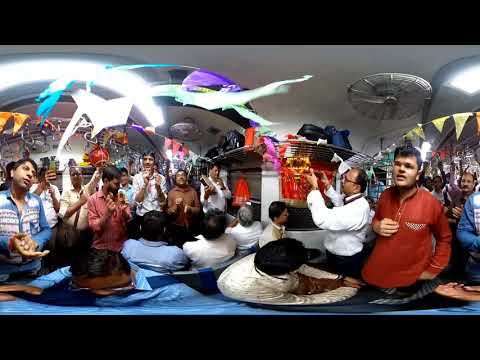The image features a distorted, fish-eye lens view of a lively gathering, possibly a celebration, that gives the impression of being taken inside a building, such as a party consignment store or a clothing store. The photo is bordered by a dark black bar across the top and bottom, each occupying about an eighth of the image. In the scene, we see predominantly dark-haired men, some of whom are distorted due to the lens effect, especially on the left and right sides of the image. Several of the men are wearing white shirts, with some sitting and others standing. A noticeable figure is a man in white with glasses, holding an object with both hands, possibly a microphone. Another individual, dressed in brown, is actively clapping. The ceiling features a circular-shaped metal fan, positioned towards the upper right of the image. Additionally, there are what appear to be paper planes floating in the air, attracting the gazes of some individuals. The decorations on the wall and the festive atmosphere, enhanced by various objects and possibly mobiles hanging in the scene, suggest a party or celebration, potentially in an Indian setting.